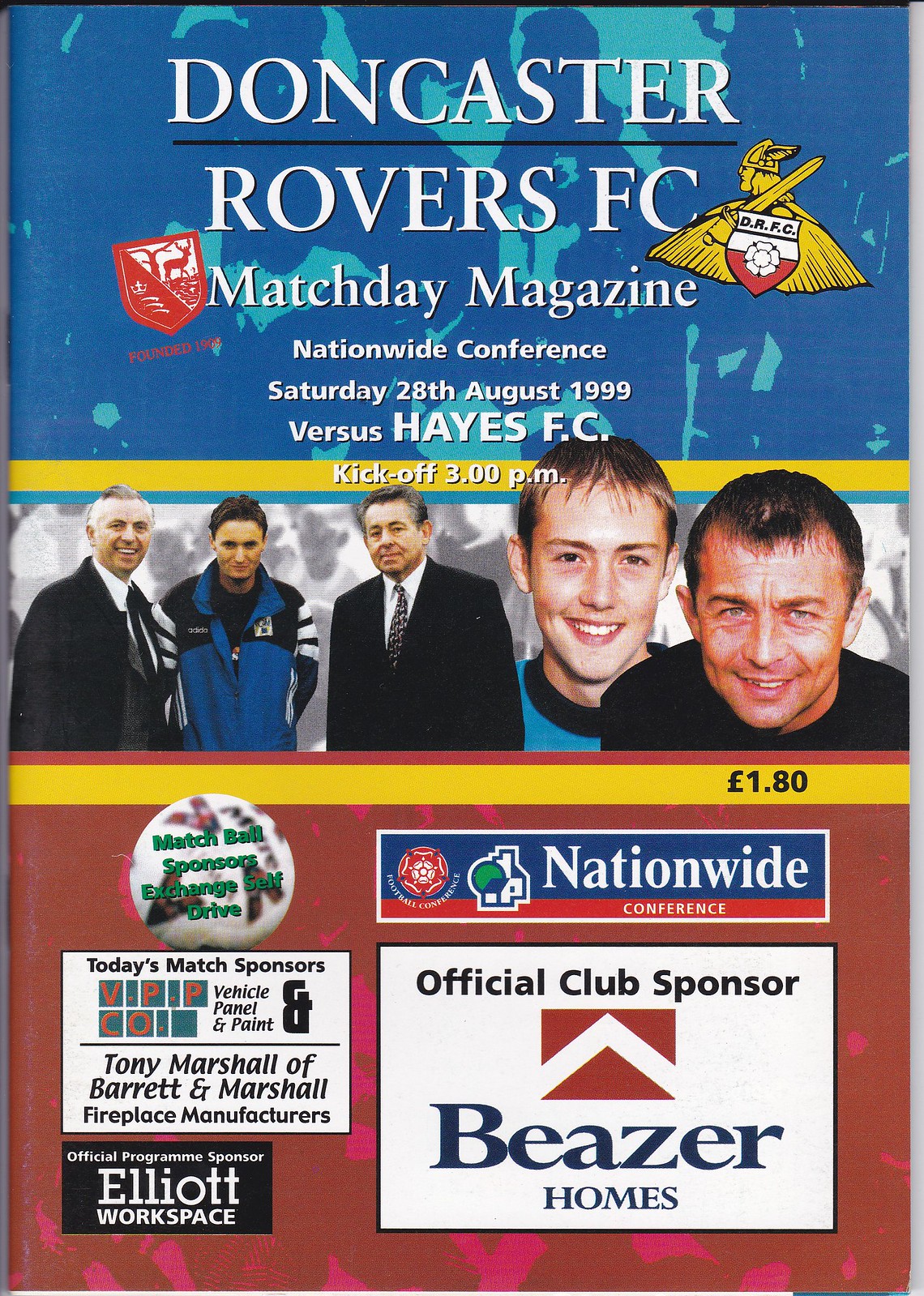The cover of the Doncaster Rovers FC Matchday Magazine for the Nationwide Conference match against Hayes FC, scheduled on Saturday, August 28, 1999, at 3 p.m., is a vibrant and detailed composition. The top section features a background of blue and green hues. Central to the image are five males, likely comprising managers, the team captain, and players, positioned between the top and bottom sections. The first three individuals are depicted in half-length photos, while the last two are headshots. A yellow bar beneath the group prominently displays the price of £1.80. The lower section of the cover, against a red background, includes a soccer ball graphic and text mentioning 'Match Ball Sponsors Exchange Self-Drive' and 'Nationwide Conference'. Additional sponsors highlighted are Beezer Homes (official club sponsor), Elliott Workspace (official program sponsor), and today's match sponsors VPP Co. Vehicle Panel and Paint, Tony Marshall of Barrett & Marshall Fireplace Manufacturers. A small button, whose text is not fully clear, also features to the left side of this section.